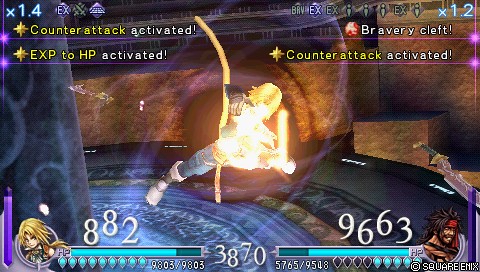This image is a screenshot from a video game, showcasing a dynamic scene set within what appears to be an underground cave or temple. The main character, positioned in the center, is engulfed in flames or glowing brightly, making it tricky to discern precise details. He seems to be airborne, possibly swinging from a rope or grappling hook, and facing off against an unseen enemy. This character might be holding a bow or a sword.

On the left side of the screen, there are several indicators and text overlays. "Counter-Attack Activated" and "EXP to HP Activated" are prominently displayed, suggesting the player has triggered special abilities. There are also numerical hit points: 882 on the left for the player's character and a significantly higher 9663 on the right for the opponent, indicating an ongoing battle. Additionally, a teal bar that depletes to gray, possibly representing health or energy, runs across the top of the screen, and there are supplemental teal markers at the bottom, which might signify lifelines or additional resources. 

The backdrop is richly detailed, with a design that evokes the atmosphere of an ancient, possibly Egyptian, tomb. The overall image is vibrant and striking, with various colors and lights enhancing the dramatic conflict taking place. A copyright notice is faintly visible at the bottom of the screen, suggesting ownership of the game's content.